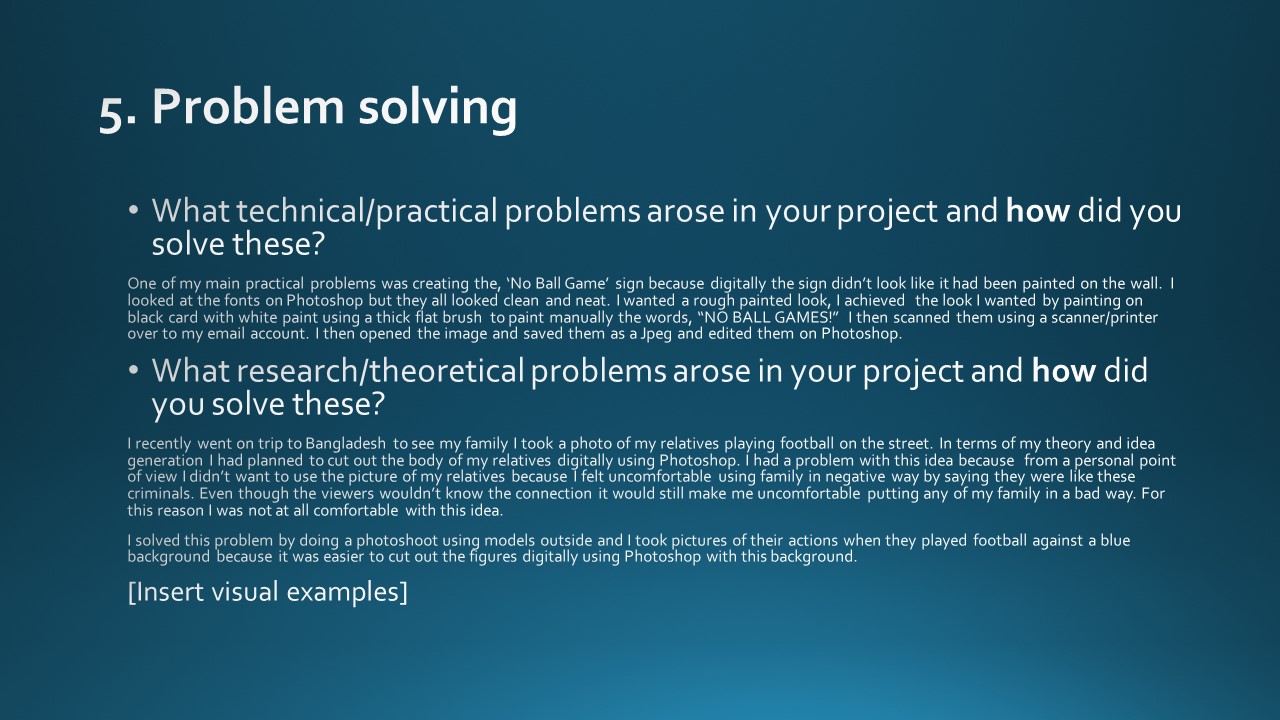The image appears to be a slide with a blue background, slightly darker at the top and lighter at the bottom. The text is all in white. At the top, in large text, it says "5. Problem Solving." Below the title, there are two sections, each with a heading in larger font followed by smaller text. 

The first section is titled "What technical/practical problems arose in your project and how did you solve these?" The text that follows describes a problem with creating a digital sign that looked painted. To solve this, the individual painted the sign manually on black card with white paint, scanned it, and edited it in Photoshop.

The second section is titled "What research/theoretical problems arose in your project and how did you solve these?" In the smaller text, the individual recounts a trip to Bangladesh where they took photos of relatives playing football. They initially planned to use these images in their project but felt uncomfortable portraying their family negatively. To resolve this, they conducted a photo shoot with models against a blue background, which made it easier to digitally edit the photos in Photoshop.

At the bottom of the slide, in larger font, it says "Insert visual examples."